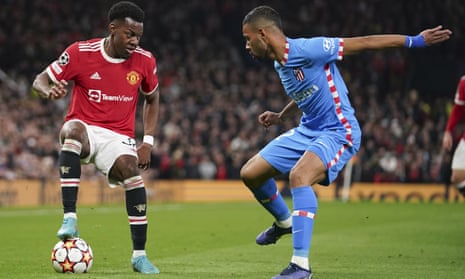The image captures an intense moment in a soccer match, professionally taken with a sharp focus on the athletes and a blurred backdrop of a massive crowd, hinting at an outdoor event. The central figures are two African-American players. The player on the left sports a dark skin tone and short, poofy hair. He’s donned in a light cranberry red jersey with white accents, likely team sponsors, text not legible. His outfit includes white shorts and knee-high black socks with white stripes, completing his look with light blue cleats. With a determined gaze, he places his right foot on a vibrant soccer ball adorned with yellow, red, and blue stars, while his left foot is firmly planted on the grass.

Opposing him is a player with a dark skin tone in a baby blue ensemble – a jersey, armband, shorts, and knee-high socks, accentuated with red and white details. His dark blue cleats contrast against his uniform. This player has his left foot on the ground, his right foot raised, and his left arm extended straight behind. The background reveals a packed stadium with hundreds of fans and a faint brown fence, reflecting the vibrant and competitive atmosphere of the match.